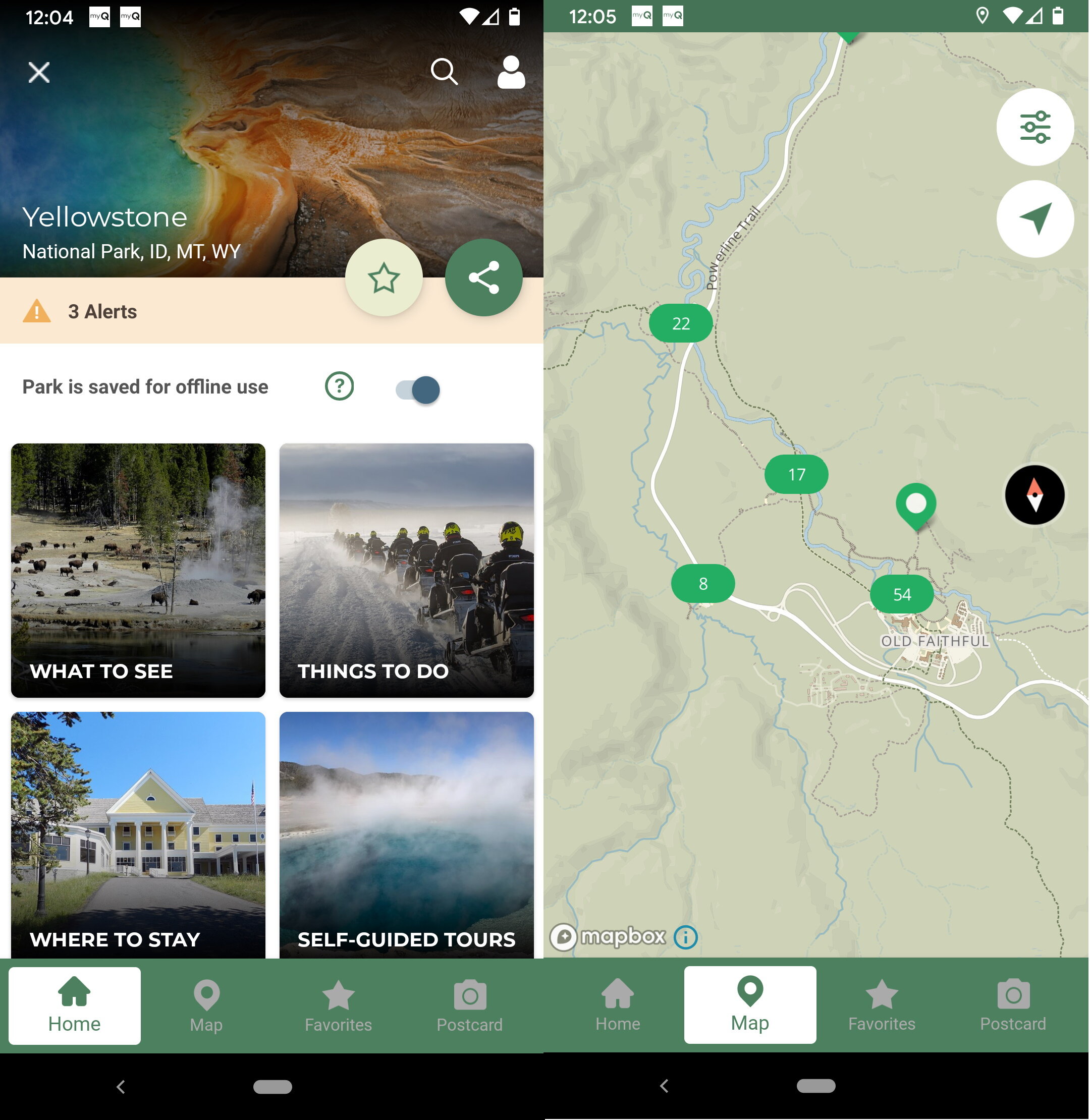The first screenshot displays the time at 12:04 PM, with visible icons in the top right corner indicating a connected WiFi network, strong signal strength, and the current battery level. 

The second screenshot, shown to the right, has the time at the top left corner reading 12:05 PM. This image also displays several icons, including location status, WiFi connection, network signal indicator, and battery level.

Within the first image on the left, there is a detailed navigation screen for Yellowstone National Park. The display includes street alerts and confirms the park is saved for offline use. Options presented are 'What to See,’ ‘Things to Do,’ 'Where to Stay,' and 'Self-Guided Tours.' 

The second image on the right showcases specific points of interest within Yellowstone, including 'Old Faithful' and 'Powerline Trail.' Also visible are filter options, FIWO (likely referring to 'Find What’s Open') rights, a postcard feature, and the home icon for returning to the main navigation.